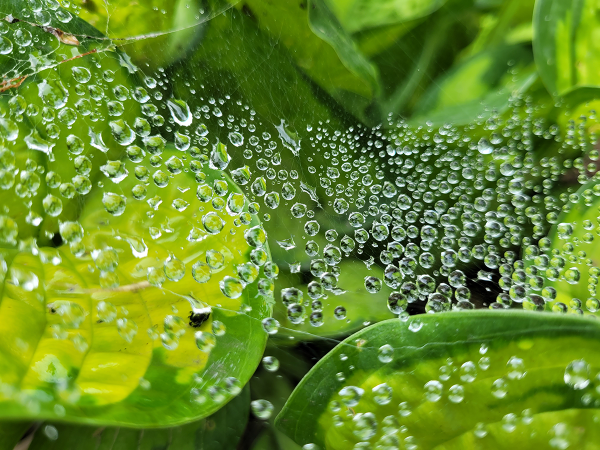The image vividly captures a realistic, high-definition close-up of lush green foliage, showcasing a rich tapestry of leaves in various vibrant shades of green, interspersed with hints of yellow. The photograph highlights the intricate details of a spider web that spans across the image, adorned with numerous water droplets. These droplets range from round, bubble-like formations to longer drips, each meticulously spaced along the web. The raindrops are transparent, catching the light to add an exquisite sheen. The background features more greenery, enhancing the natural, outdoor setting of the photograph. The detail and clarity suggest it could be mistaken for a computer-generated image, but the organic complexity confirms it as a skillfully captured true-to-life scene.